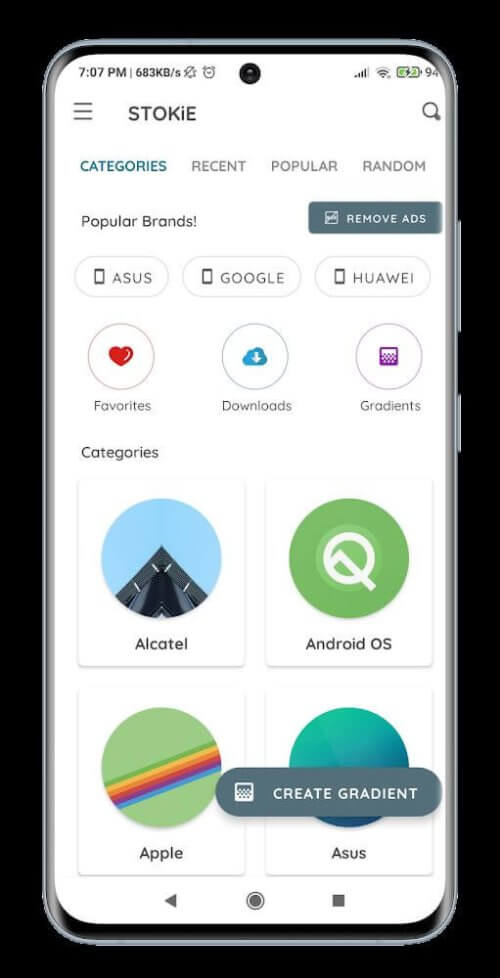The image showcases a mock-up of a phone displaying an app called 'Stokie' (with all letters capitalized except for the 'i'). The app interface resembles an app store, featuring a white background and a grid layout of categories for easy navigation. At the top, users can browse different sections such as 'Recent', 'Popular', and 'Random'. These categories include diverse brands like Alcatel, Android OS, Apple, and Asus, each represented with an illustrative image; for instance, Apple features an abstract rainbow design, while Alcatel displays an upward view of a building.

Additional user interface elements include buttons for 'Favorites', 'Downloads', and 'Gradients'. Interestingly, there is also an option to 'Create Gradient' located at the bottom right of the screen, though its functionality isn't entirely clear. The app appears to be geared towards phone shopping, potentially allowing for both new and used items, offering a visually engaging and organized shopping experience.